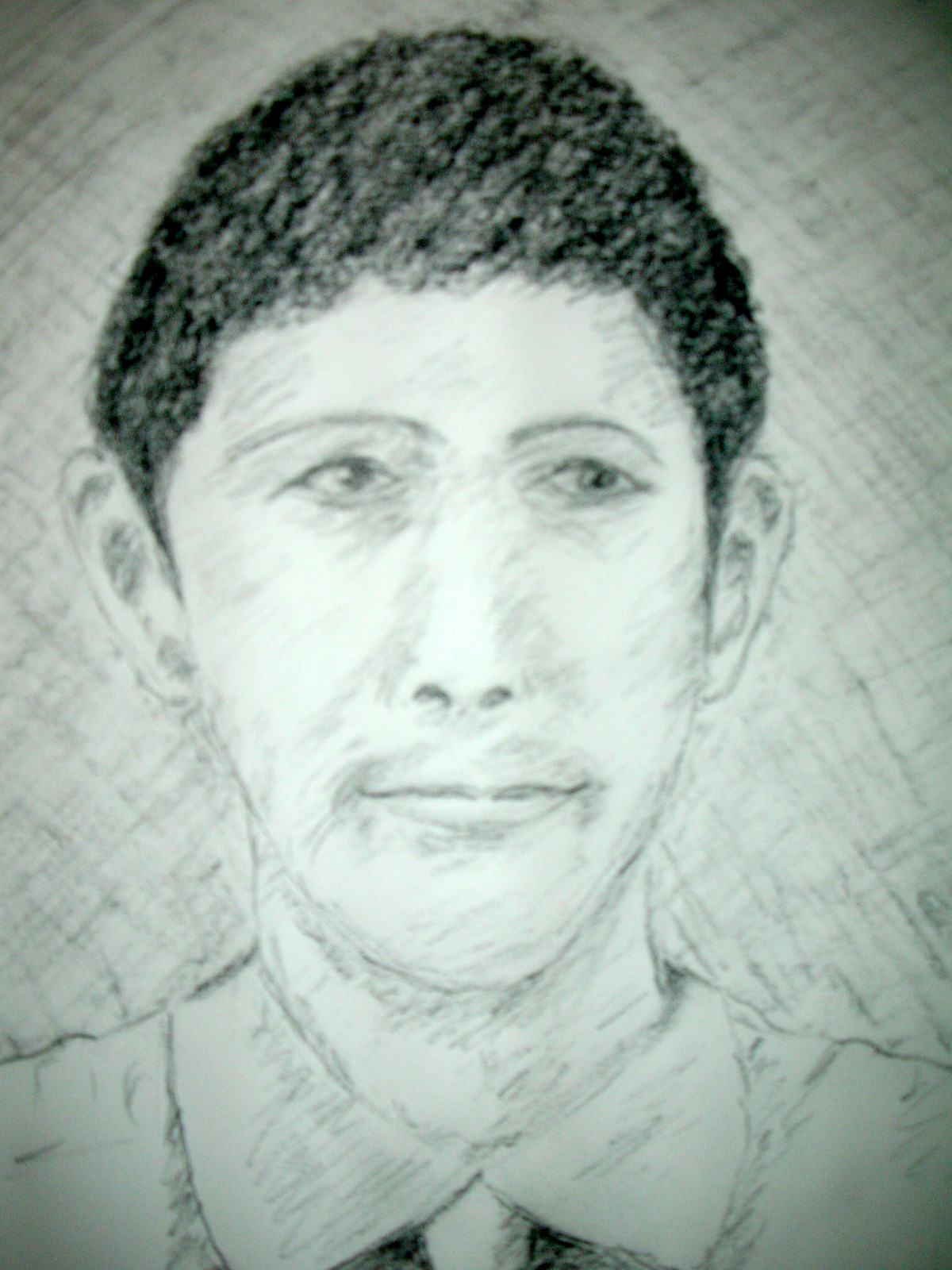The image depicts a detailed pencil sketch of a person with distinct facial features and attire. The head appears effeminate, framed by a short afro hairstyle. The person has prominent, large ears and expressive, thick eyebrows. Their lips are full, and they possess a broad nose. The background of the image is filled with abstract scratch marks, adding texture to the composition.

The individual's outfit includes a collared shirt, with a tie that is visibly marked with black streaks on the left side. The ears are shaded in black, providing contrast and depth to the sketch.